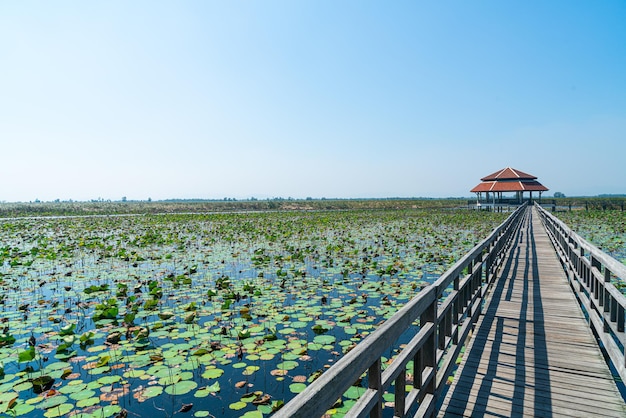This photograph, taken on a clear, sunny day with a cloudless sky, captures the serene beauty of the Khao Sam Roi Yot National Park in Thailand. Dominating the center of the image is a light blue-gray wooden walkway, featuring modest railings that guide your gaze toward a distant pavilion. This distinctive pavilion, with its two-tiered hexagonal roof in a vibrant red-orange hue, stands prominently on the right side of the frame, about halfway into the picture. The walkway and pavilion are set against a background of calm, still waters, the surface of which is almost entirely covered with lily pads and lotus leaves, giving the scene a lush, green texture. 

The lake, extending to the left side of the photograph, is framed by a handful of barely visible tall buildings on the distant horizon, shrouded in a light haze. The sky transitions smoothly from a light white near the horizon to a deeper blue at the top right of the image, enhancing the ethereal quality of the setting. The absence of visitors and the lack of blooming flowers add to the tranquil, undisturbed atmosphere of this natural landscape, making it a captivating representation of this national park’s picturesque allure.